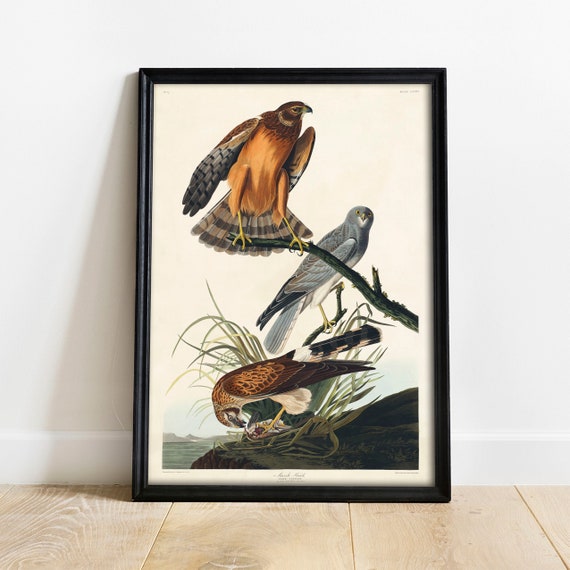This image is a photograph of a framed artwork depicting three birds of prey, presumably falcons or hawks, rendered in a detailed, colored drawing style. The frame is a black wooden one, with the artwork leaning against a bright white wall atop a light wooden floor. The scene within the artwork is primarily white but includes elements of a natural habitat, such as a dirt bank with water at the bottom and mountains in the distance.

At the top of the image, perched on a branch, is a large bird with an orange-brown underbelly and dark gray feathers on its wings. Its short, hooked beak suggests it is a raptor. Below it, centered in the composition, another bird with gray plumage and black tail feathers sits on a different branch. This gray bird shares similarities with the first bird, suggesting it could represent the female of the species. At the bottom, on what appears to be the shore of a body of water surrounded by tall grass and vegetation, a third bird with a golden-brown plumage is depicted eating something, possibly a lizard. The artwork, meticulous in its detail, reveals aspects of the birds' nesting behavior and habitat.